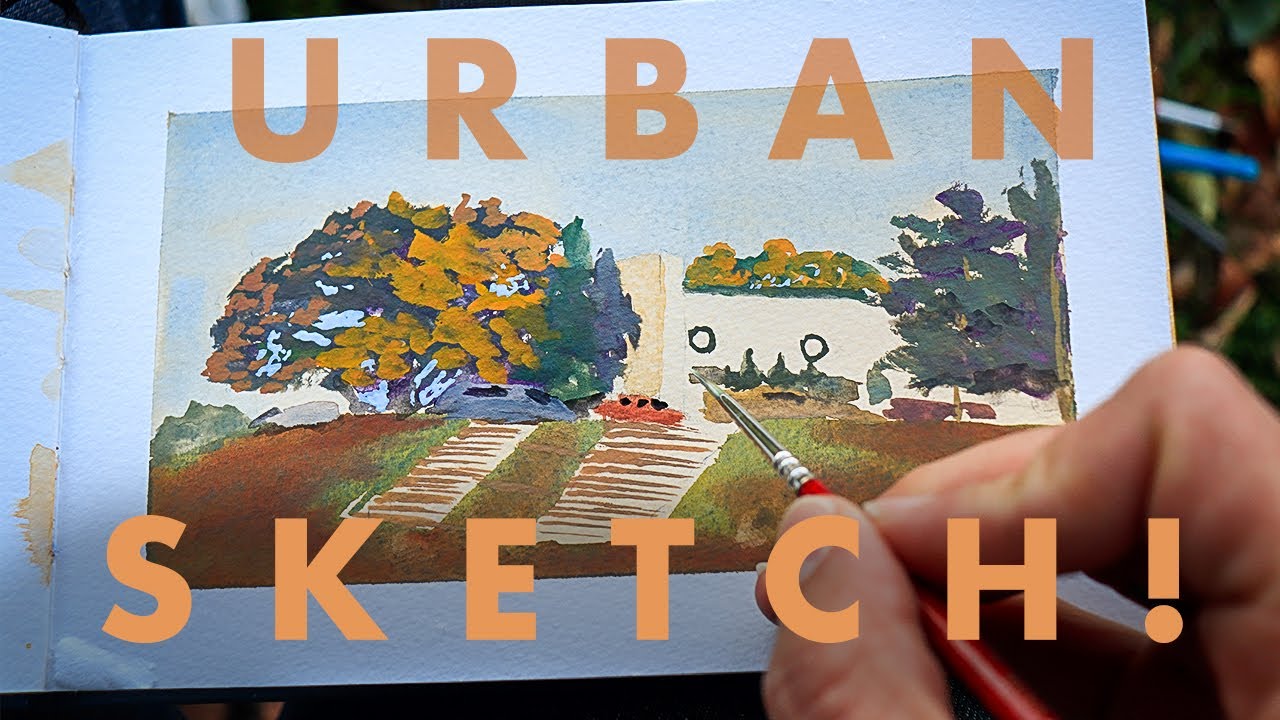The detailed image captures an indoor close-up of an artist's hand holding a fine-tipped red paintbrush with a silver tip, poised over a small sketchbook with white paper. The sketchbook features an intricate watercolor painting of a landscape, showcasing a house on a slight mound with steps leading up to it. The scene includes trees flanking both sides, vibrant with varying shades of green, orange, and blue, amidst a foreground of grass that transitions from green to brown. Parked near a white building are two cars, one red and one blue. The top of the sketchbook prominently displays the text "URBAN" in large, spaced-out, capital orange letters, while the bottom is marked with the word "SKETCH!" in the same style and color, emphasizing the urban sketching theme of the artwork and potentially suggesting its use as a product image for advertising the sketchpad.